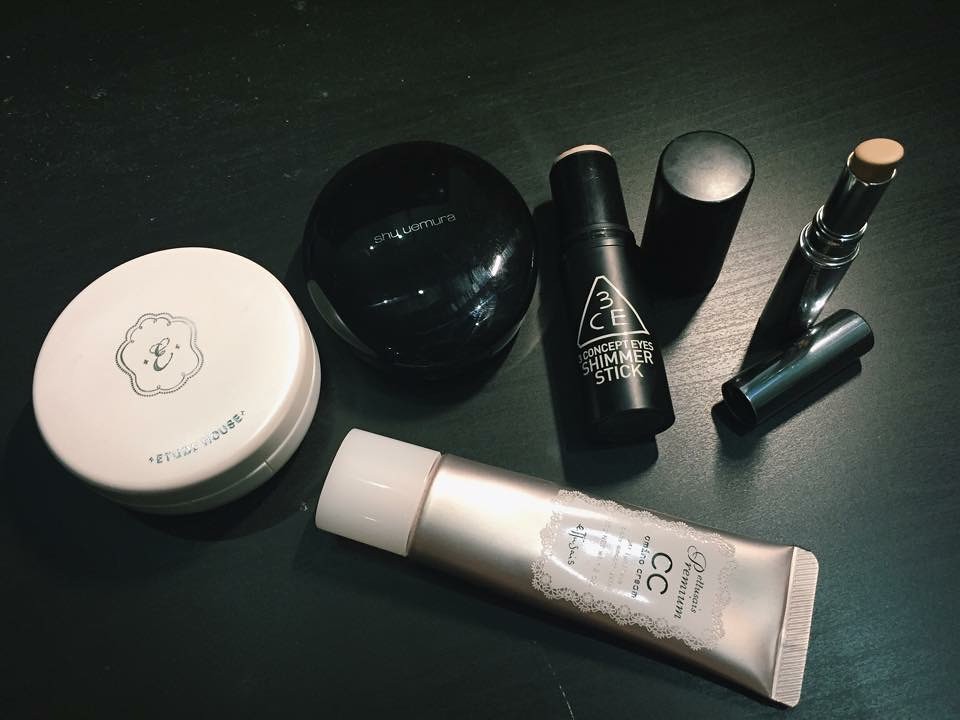This indoor photograph showcases an artfully arranged selection of makeup products on a matte black wooden surface, where the grain of the wood is subtly visible under the overhead lighting from the top right. 

On the far left, a round tub featuring an 'E' inside a decorative pattern on its lid sits, its writing smudged from years of use. Adjacent to it is another round, black object with light reflecting off its glossy surface, the brand name in white on the lid. 

Next in line is a black shimmer stick with its lid removed; the product itself, a pale creamy color, lies flat on the table next to the standing lid. The front of the shimmer stick is marked with a white triangle displaying '3CE' and further labeled as 'Concept Eyes Shimmer Stick.' 

Under the brightest pool of light, there is a shiny black lipstick container with the lid lying flat beside it, and the lipstick, in a nude tone, standing upright. 

Lastly, across the bottom of the image, a silverish tube with a white lid lies diagonally, adorned with a lacy pattern and branded with '3CE Cream' along with additional information. The packaging extends from the bottom right corner towards the center left, adding a structured yet elegant touch to the display.